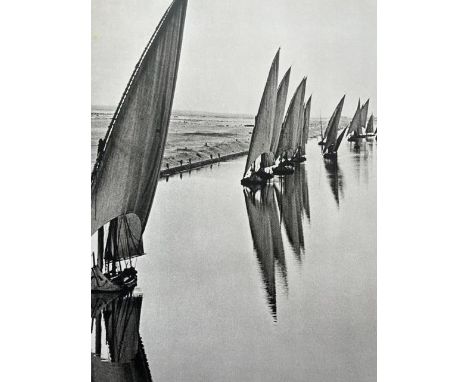This captivating, rectangular, black-and-white photograph, likely taken in the early 1900s, measures approximately two and a half inches high by one and a half inches wide. It portrays an array of sailboats lined up in a neat row. There are about eight to twelve sailboats, each featuring a tall, triangular sail perched atop a small, curved hull. These boats are positioned near a beach or a riverbank, set approximately 20 feet back from a retaining wall that struggles to hold back the ocean waves crashing over it. The still, highly reflective waters capture the mirrored images of the sailboats, extending slightly towards the upper right corner of the composition. The sky above is a clear, undisturbed gray, providing a stark yet harmonious backdrop to the serene yet dynamic scene below. The land in the distance merges seamlessly with the hard-packed dirt embankment, adding depth and context to the historical and atmospheric essence of the image.